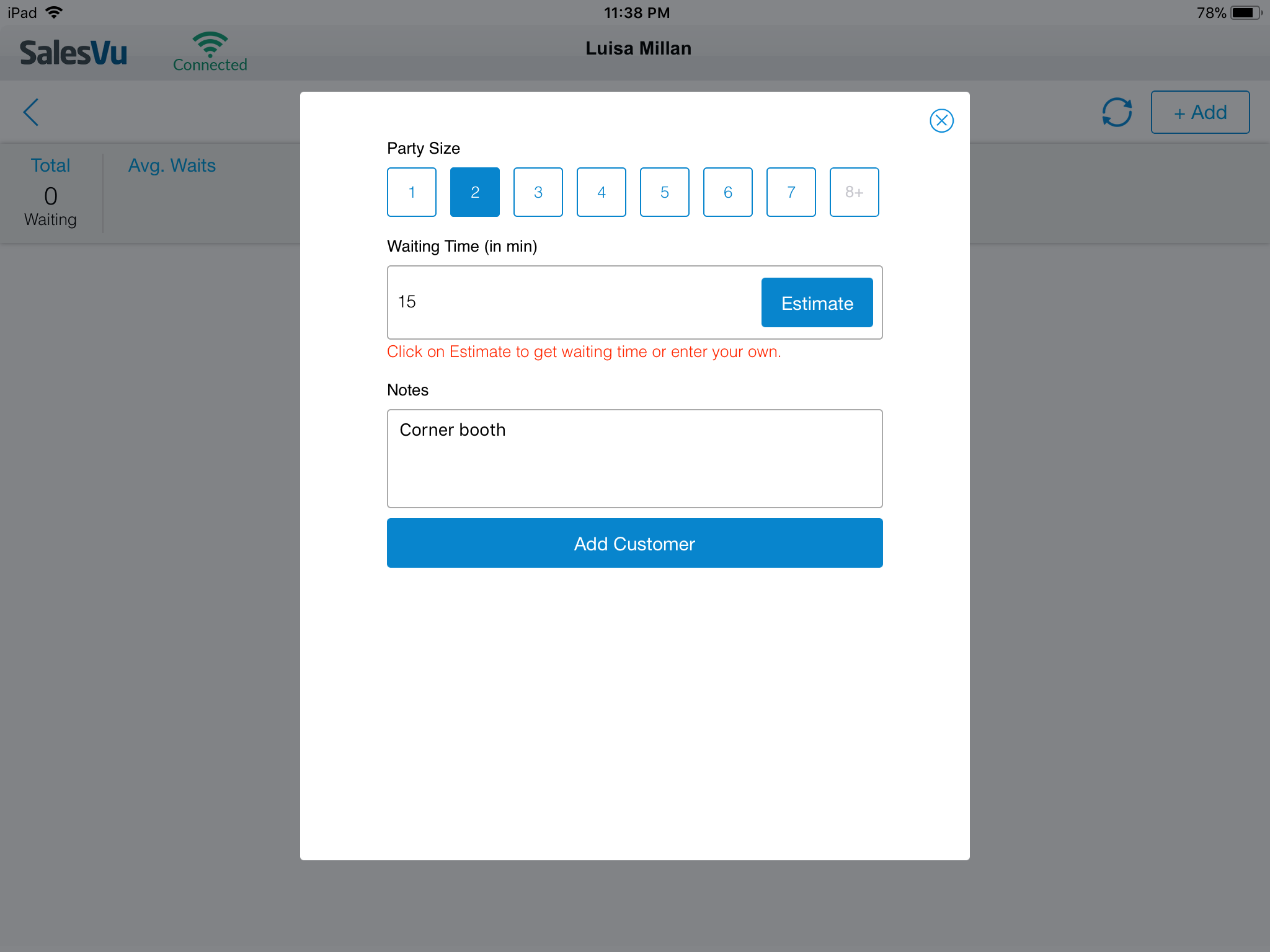**Detailed Caption for the Screenshot of a Restaurant Reservation System**

This screenshot captures the user interface of a restaurant reservation system viewed on an iPad. A prominent white overlay dominates the center of the screen, presenting options and details related to a customer’s reservation.

At the top of the overlay, the "Party Size" section displays numbers 1 through 8+, each boxed within a blue square. The number 2 box is highlighted, indicating the selected party size. Just below, there is an entry box labeled “Waiting Time” with a specified estimate of 15 minutes. Adjacent to this, a clickable “Estimate” button is visible. The following section, titled “Notes,” includes an input box containing a note that the customer requests a corner booth.

The main page, partially obscured by this overlay, features various elements. In the upper left corner, the section labeled “Sales View” is visible, and above it, the word “iPads” appears. Indicating a secure connection, the Wi-Fi symbol is accompanied by the word “connected.” At the top center of the screen, the customer’s name, "Louisa Milan," is prominently displayed, with the current time, 11:38 PM, positioned above it. To the far right, the battery icon shows a remaining charge of 78%.

Toward the left side, additional information can be observed. Labels “Total” and “Waiting” are present with the number zero underneath each. A section titled "Average Waits" is partially visible but further details are obscured by the overlay.

Overall, this descriptive caption thoroughly details the interface elements and functionality presented in the screenshot, providing a clear insight into the restaurant reservation system's layout and user experience on an iPad.